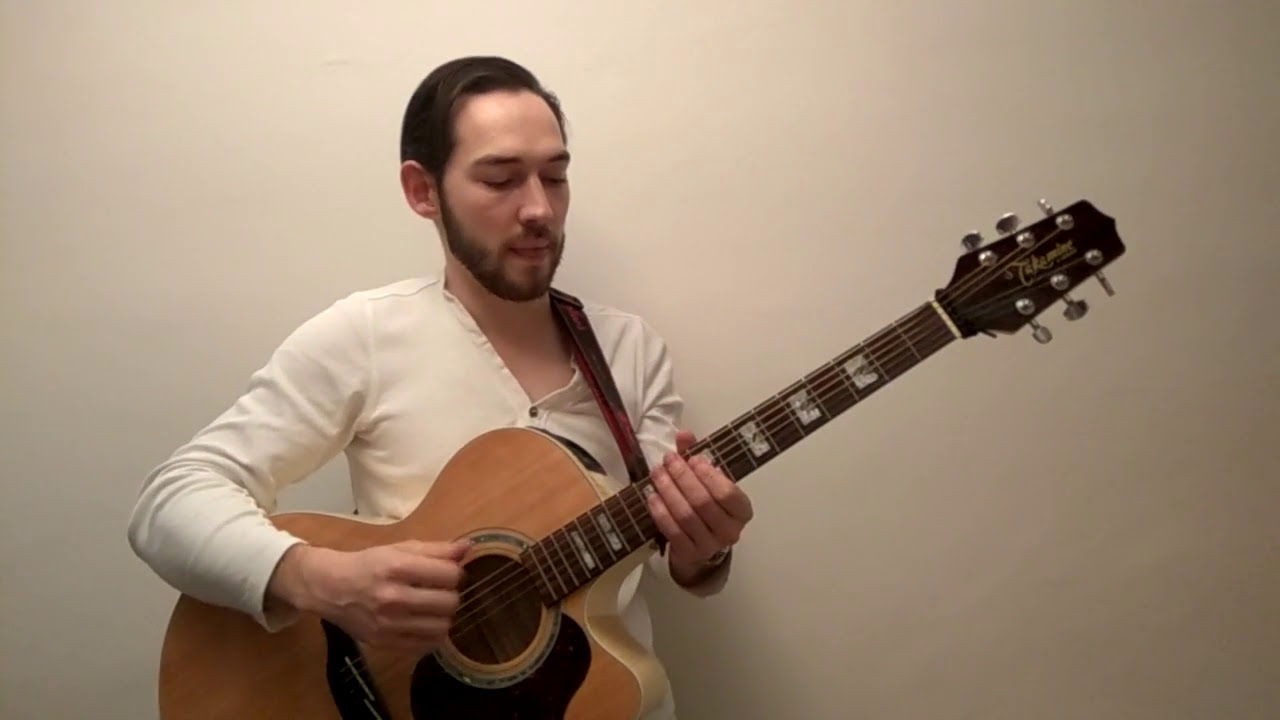This is an image of a middle-aged man, aged between 25 and 35, standing slightly left of center in the frame. He has short brown hair and a short brown beard paired with a short mustache. The man is wearing a white, long-sleeved button-down shirt and is focused intently on his guitar. He holds a wooden acoustic guitar with a light brown body, a dark brown neck, and silver tuning pegs on the black headstock. The guitar is angled upwards as he appears to be actively playing it, strumming with his right hand while his left hand manipulates the fretboard. A strap is positioned over his shoulder, aiding in his stance. The background is a white to beige-colored wall, providing a simple contrast that accentuates the man and his guitar. His gaze is directed downwards at the guitar, concentrating on the placement of his hands, emphasizing the seriousness of his play.